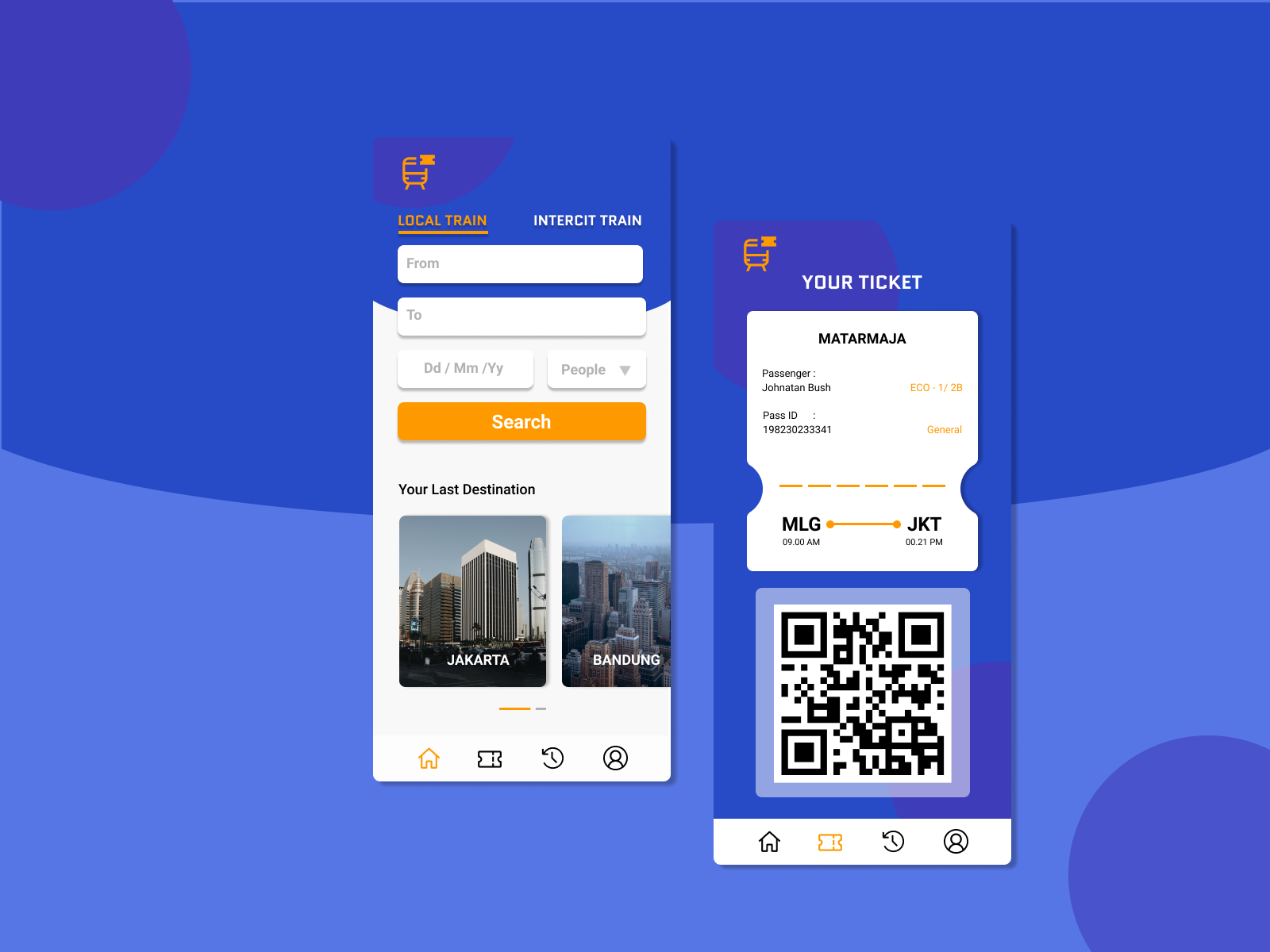The provided image is a screenshot featuring two distinct sections that depict the interface of a train booking application. The first section showcases options for selecting either a local train or an interstate train (abbreviated as I-N-T-E-R-C-I-T), accompanied by text boxes for inputting departure and destination locations. Additional boxes are formatted for date entries, using a structure of two D's, two M's, and two Y's to indicate day, month, and year respectively. Below these boxes are fields for entering the number of passengers and other relevant details. A prominent orange rectangle with the label "Search" is also visible, designed to initiate the search process for available trains.

The second section adds more depth, displaying what could possibly be personalized results or settings. It includes a line mentioning "Your last destination" and "My trauma Josh M-A-T-A-R-M-A-J-A," perhaps indicating previous trips or user-specific information. There are icons representing various functionalities: an orange train in the top left corner, an orange house, a ticket symbol, a reverse symbol possibly indicating a return trip, and a profile symbol on the first screenshot. The second screenshot repeats similar icons but highlights the ticket symbol in orange, and rearranges the icons including a house, the ticket symbol, the reverse symbol, and the profile symbol, potentially implying a different section or state within the app. 

Thus, the image provides a comprehensive glimpse into train booking options with detailed user interface elements, enhancing efficiency for travelers managing their journeys.